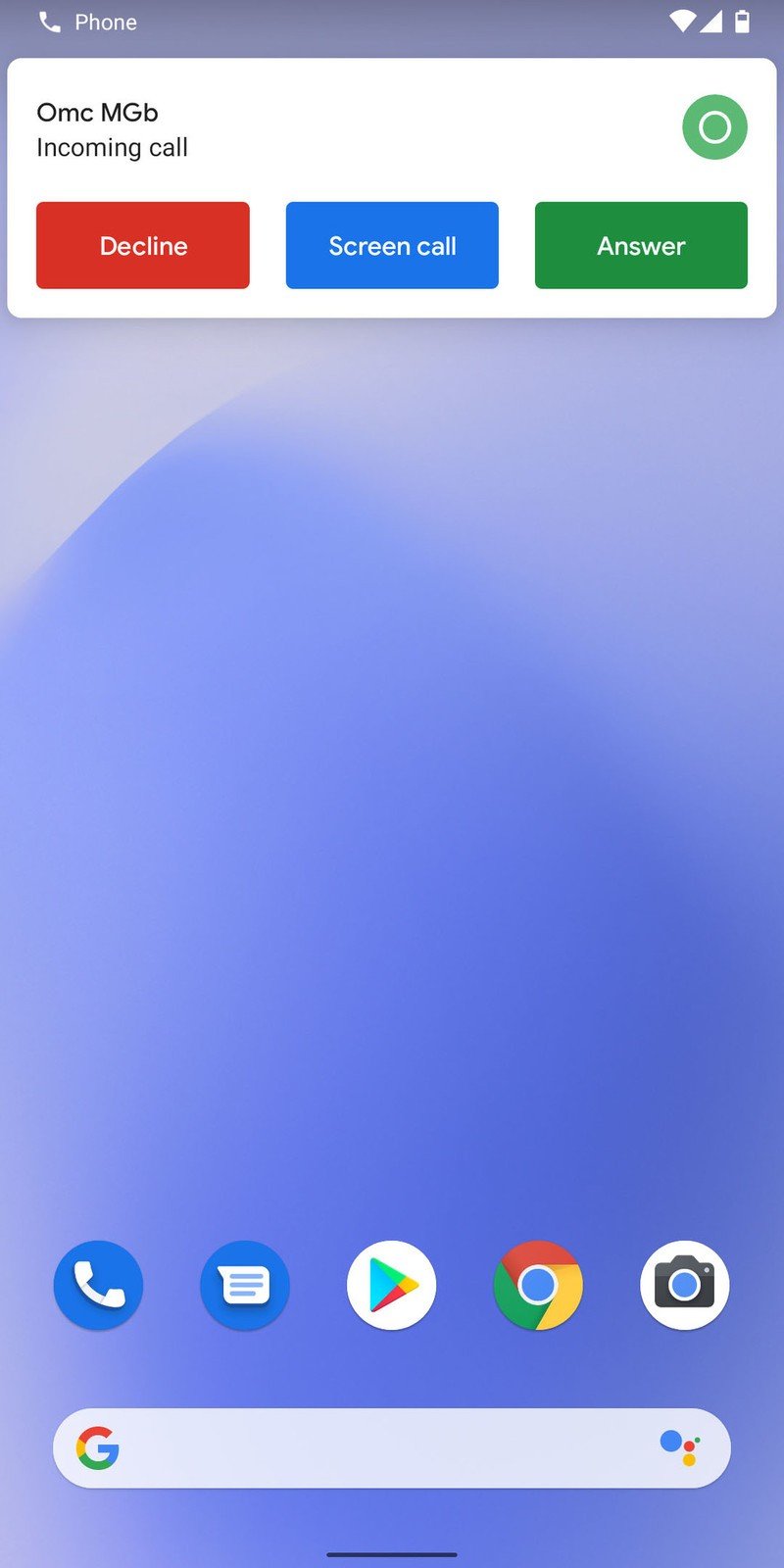This is a detailed screenshot of a mobile phone's home screen. The background features a gradient ranging from a lilac hue in the center to a lighter purple at the top. In the upper left corner, there's a white phone handset icon labeled "Phone." The upper right corner displays white icons for Wi-Fi, mobile signal, and a half-filled battery.

Below these icons, a white pop-up rectangle with black text reads "OMC MGB Incoming Call." Beneath this notification, there are three response options: a red rectangle with white text that says "Decline," a blue rectangle with white text that says "Screen Call," and a green rectangle with white text that says "Answer." Additionally, a green circle containing a white circle is located in the upper right section of this pop-up.

At the bottom of the screen, the home screen displays five icons for essential applications: Phone, Text Messages, Google Play Store, Chrome, and Photos.